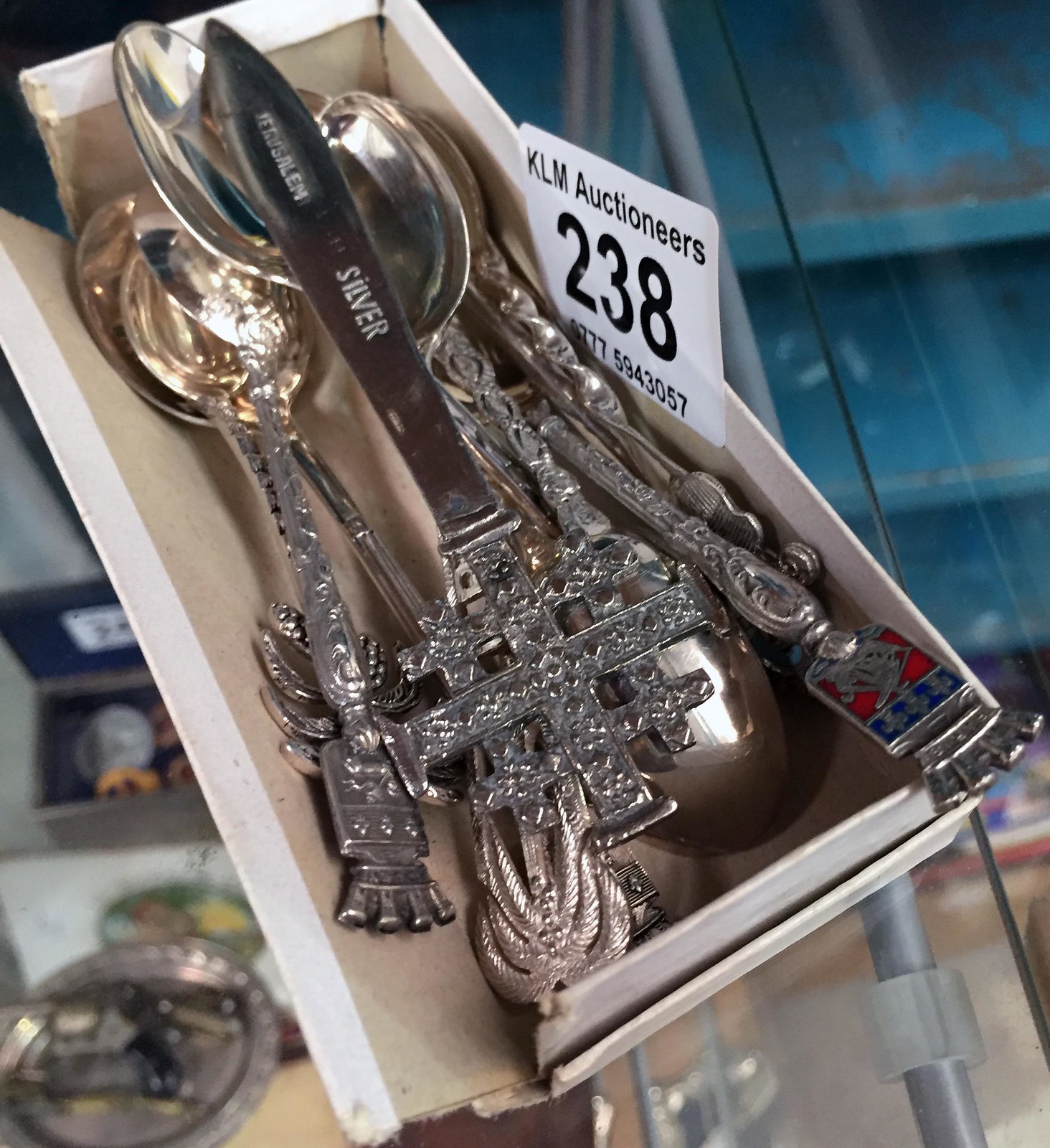In this image, an overhead view captures a white cardboard box with the bottom left corner ripped on both the side and the top, revealing the beige-colored interior. Inside the box lies an assortment of antique silverware, including several souvenir spoons and a distinctive silver knife. The knife is decorated with a silver cross on top surrounded by four smaller crosses, and the blade is inscribed with the word "silver." Among the spoons, one features red and blue accents. The box bears a label reading "KLM Auctioneers 238," followed by a series of additional numbers beneath this identifier. The box is placed on a clear glass table, hinting at a display setting possibly within an antique shop, auction house, or estate sale. The background scene, seen through the glass, is out of focus, providing no specific detail.